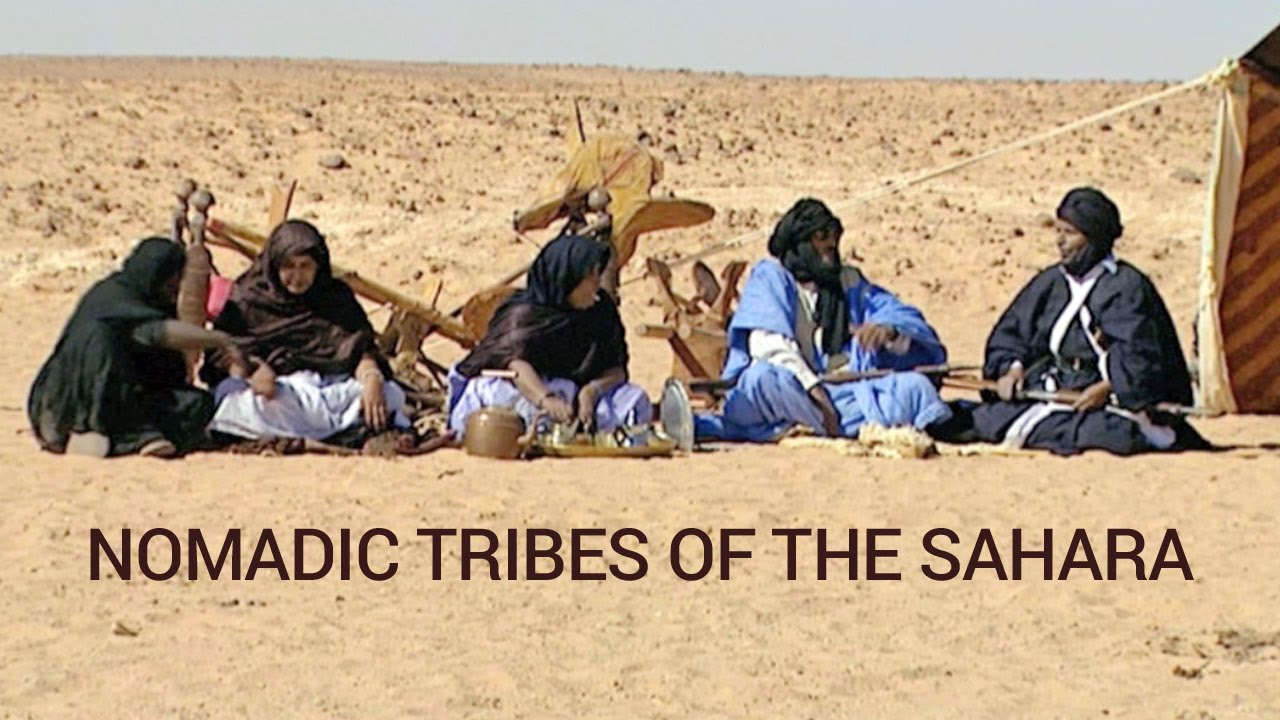In this low-resolution photograph titled "Nomadic Tribes of the Sahara," a group of five people, consisting of three women on the left and two men on the right, is seated on the desert floor. They are dressed in traditional clothing with turbans and robes, the women in headscarves and the men in turban-style headwear. A tent is partially visible to the right, with a rope extending from behind them to some wooden equipment, possibly including a wooden bucket. The desert landscape behind them stretches out endlessly, rocky and barren under a gray sky. The color palette of the image is dominated by shades of brown and black, interspersed with hints of white, blue, and a touch of pink. The scene is both serene and stark, capturing a brief moment in the vast expanse of the Sahara.